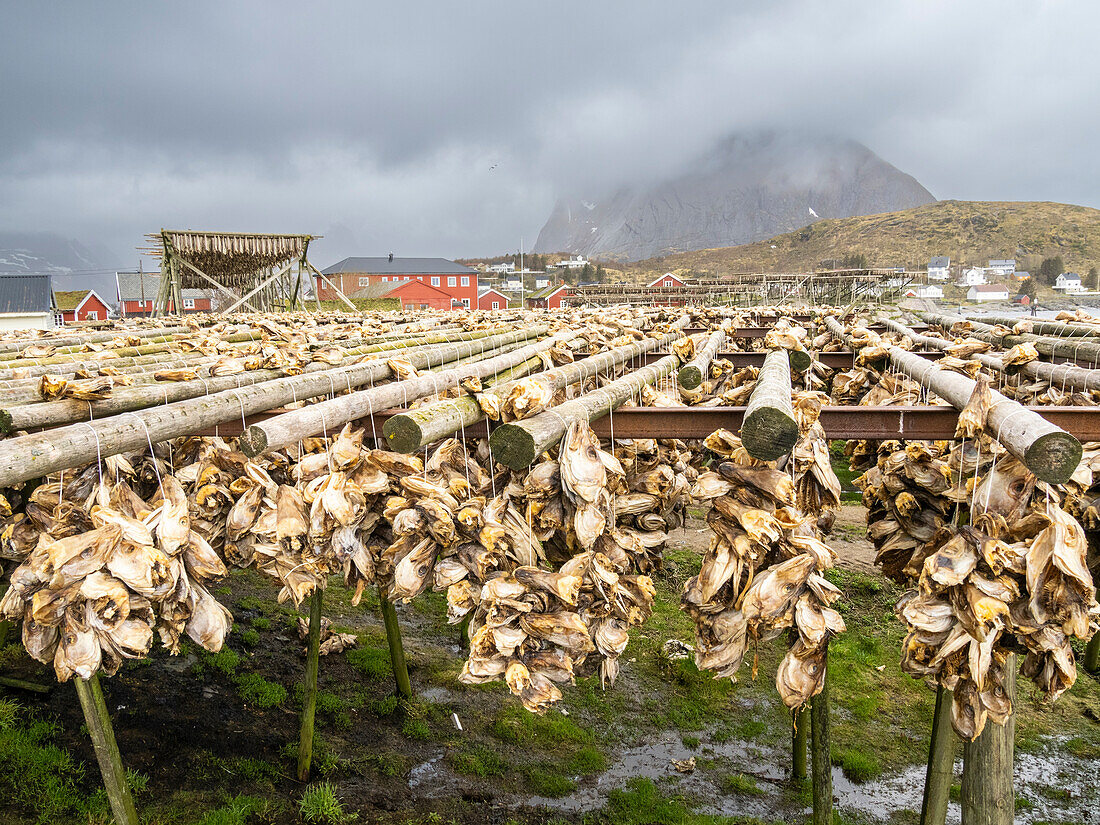The square, full-color photograph captures an outdoor farm scene during an overcast daytime, with natural light illuminating the setting. The sky is heavily clouded, contributing to a foggy atmosphere that suggests a high elevation. Central to the image is a series of wooden poles, which are laid out horizontally on metal beams, with various food items or possible vegetation hanging to dry. The ground beneath them appears wet and green, adding to the earthy tones of the scene.

In the midground, right of center and towards the top, a rounded landmass, potentially a mountain, is partially obscured by fog. On the center right stands a brown hill, and scattered across the landscape are several white houses. Just left of center, a collection of red buildings catches the eye, including a notably large barn-like structure with an awning, as well as another red building and a final white building toward the far left.

The photo also features an array of logs lying on the land, contributing to its rustic and agricultural atmosphere. The composition and placement of these elements create a serene yet somber mood, enhanced by the color palette of gray, light gray, tan, yellow, light brown, brown, and dark green. The photograph provides a detailed glimpse into a peaceful farm area set against a dramatic, cloud-covered backdrop.